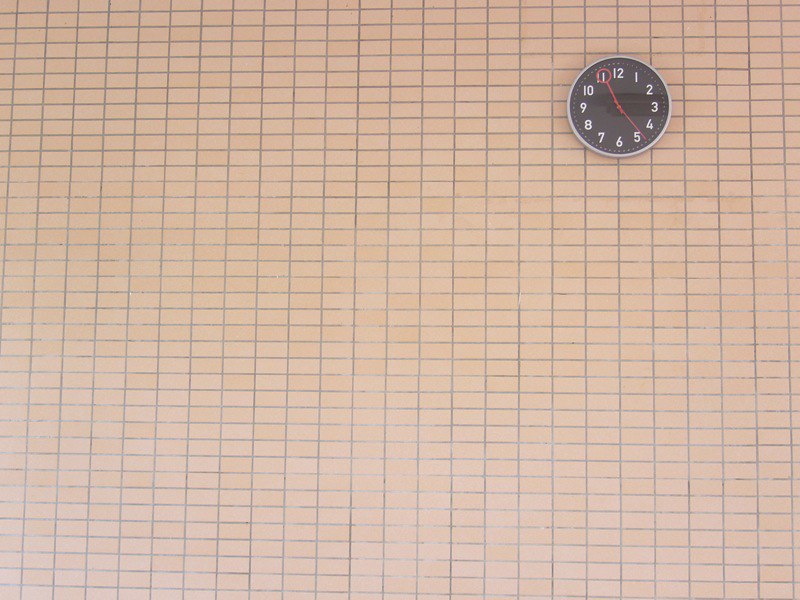This photograph captures a clock mounted on a tile-covered wall. The wall features a meticulously arranged grid pattern of small, square, tiles in shades of pinkish-red and tannish-orange, with distinct dark gray grout lines separating each tile. The carefully aligned tiles create an unbroken texture across the entire surface, which appears slightly worn and faded towards the bottom.

Centrally positioned high on the wall is the only object in the scene: a clock. This clock has a striking black face with bold white numbers running from 1 to 12, accentuated by a silver rim. Among the clock's notable details are two distinct red hands marking the hours and minutes, and a notable red circle prominently around the number 1. The clock reads 11:25, its bright red hands adding a vivid contrast against the dark background.